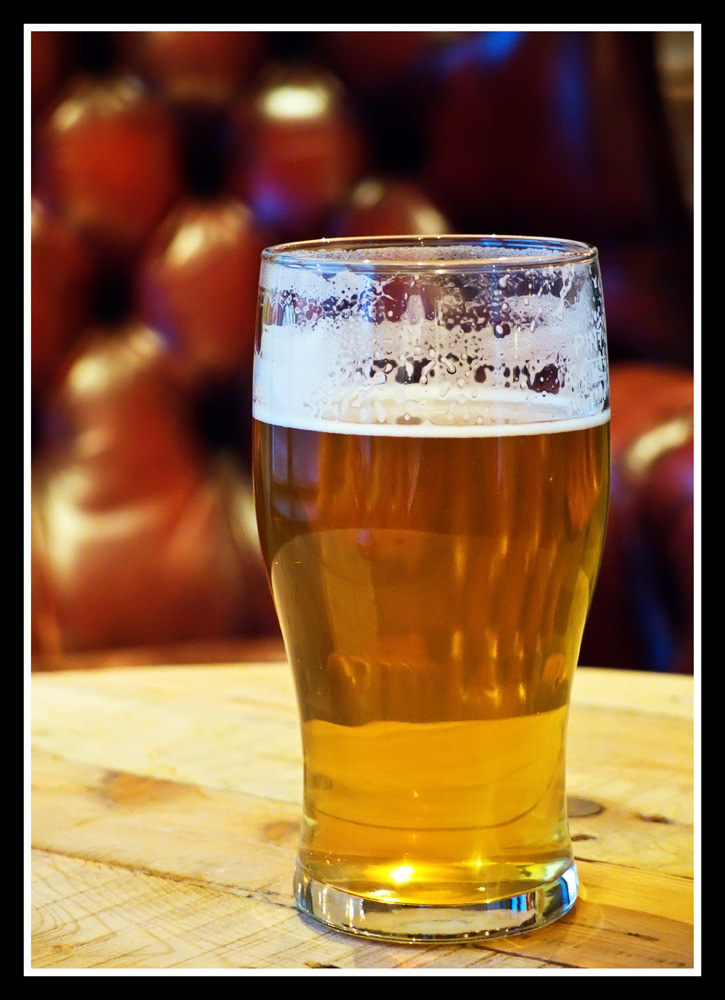This photograph, rectangular and taller than it is wide, is bordered with a thick black frame surrounding a thin white inner border. The close-up image centers on a clear glass of beer, filled to about three-fourths of its capacity. At the top of the beer, a layer of white frothy foam lingers, with traces of it clinging to the inside of the glass. The glass itself stands on a light beige, circular wooden table, which appears a bit rough and natural, rather than stained. The background behind the beer is out of focus, but faint hints of a brown leather surface, possibly the armrest of a chair or couch, are visible on the right side of the image. Overall, the photograph emphasizes the detailed textures and colors of the beer and the table, while the blurred background suggests a warm, homely setting.